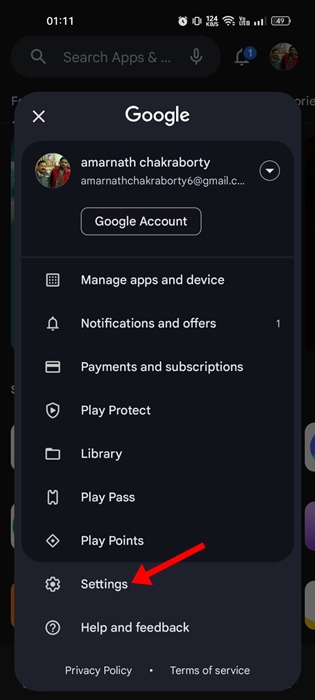This image is a screenshot taken from someone's camera display. At the top of the screen, the time is recorded as 1:11 AM, while a row of icons extends from nearly the center of the screen to the far right. Among these icons is a battery symbol showing a 49% charge. Below this, there is a search bar labeled "Search apps…" accompanied by a magnifying glass, a microphone icon, and a notification bell with a count of one. Additionally, a profile picture is visible, indicating a logged-in user.

Further down the screen, a new section appears, featuring a close button (X) and the word "Google." Beneath it, the name "Amarnath Chakraborty" is displayed, indicating the active Google account. A red arrow at the bottom points horizontally across the page towards the word "Settings," which is positioned beside a gear icon. Along the left side of this section, various options each accompanied by icons such as gears or bells are visible, with their corresponding descriptive text displayed to the right. The overall layout and elements suggest navigation within a settings or account management interface on a digital device.